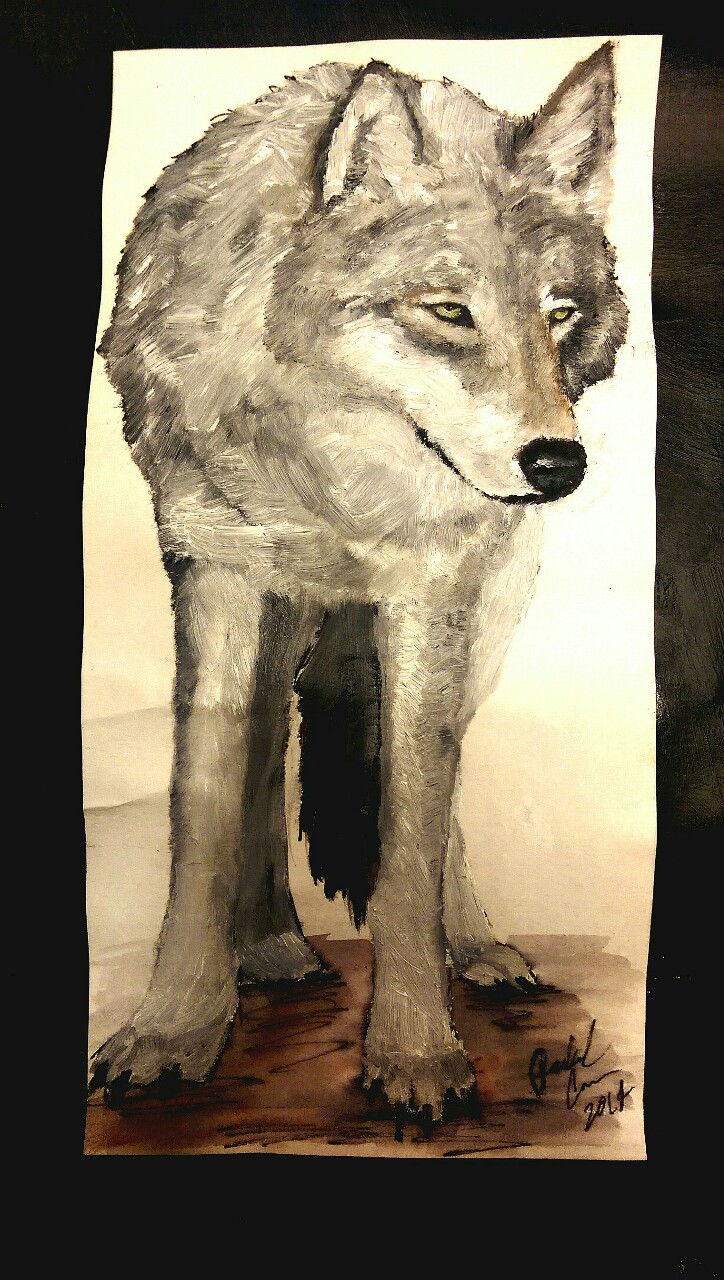The rectangular image, approximately six inches tall and two to three inches wide, is framed by a black border. Inside, the artwork portrays a gray wolf with long legs and a rounded body. The wolf, facing forward with its head turned to the right, has a black nose and yellowish eyes. Its tail, painted black, droops down between its legs. The ground beneath the wolf, rendered in reddish-brown and dark earth tones, includes shadow elements that suggest a textured, shadow-cast surface. The background of the painting features a gradient from darker hues at the bottom to a bright white at the right-hand center, transitioning to a more yellowish tone above and on the left. The wolf's pointed ears have dark gray outlines, and its black nails are visible. The artist's cursive signature is located at the bottom right-hand corner, beside the date 2014, though the name itself is difficult to discern. The painting's medium appears to involve watercolor or potentially oil, evidenced by visible brush strokes. The wolf exhibits an uninterested expression, enhancing the detailed realism of this signed 2014 artwork.